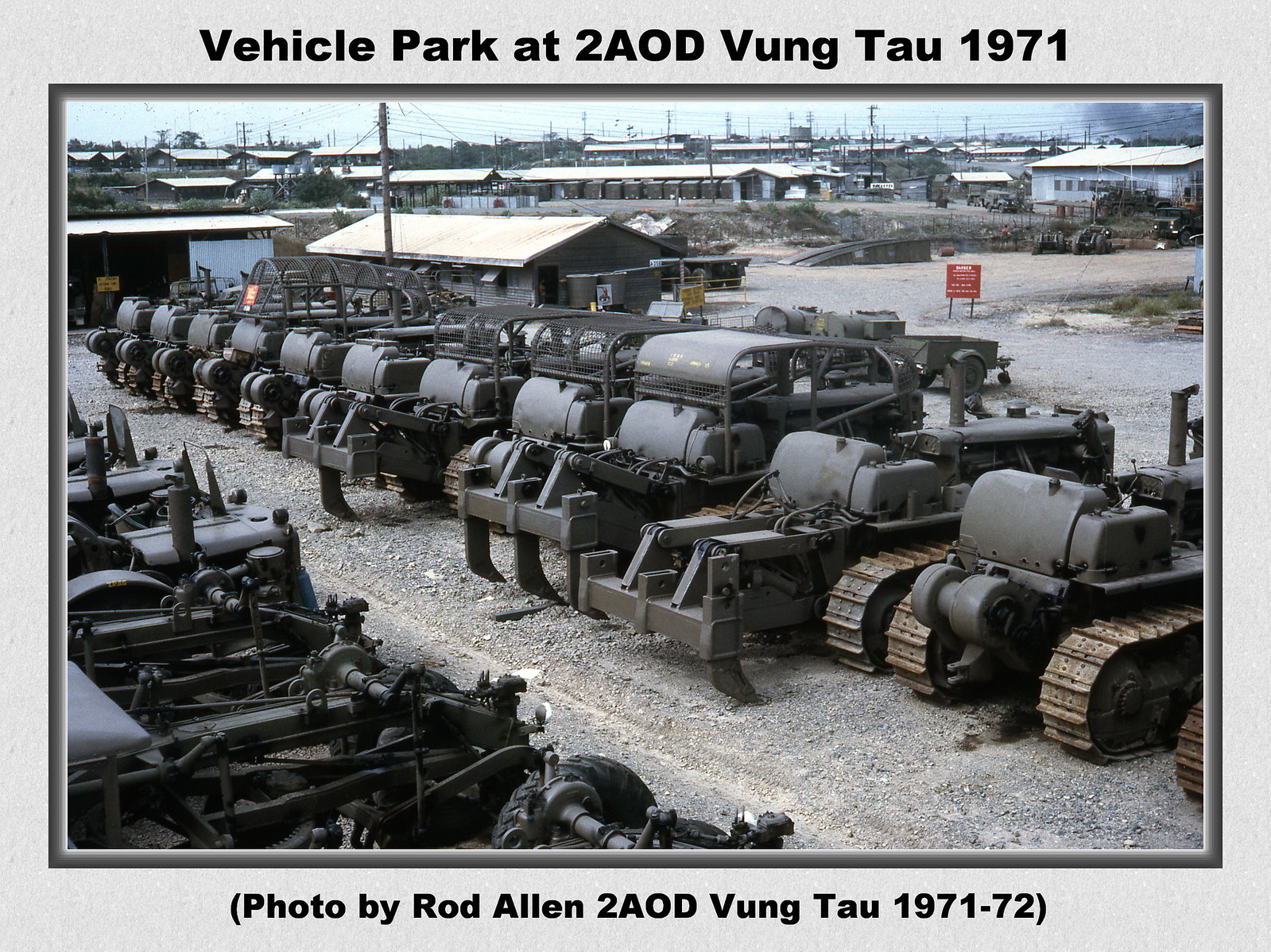The image, titled "Vehicle Park at 2AOD, Vung Tau, 1971," and photographed by Rod Allen during his service from 1971-72, depicts an outdoor scene bathed in natural daylight. The focal point is a lineup of military vehicles, possibly tanks or caterpillar machinery, organized neatly on a gravel parking lot. These vehicles are set against a backdrop of gray warehouse buildings with metal roofing, contributing to a utilitarian, somewhat industrial appearance. Scattered around the periphery are signs of life and utility: homes, telephone poles, power lines, and trees. A solitary red sign punctuates the otherwise muted color palette. The scene captures a slice of military life at an apparent base, with sheds and old machinery underscoring its functionality.